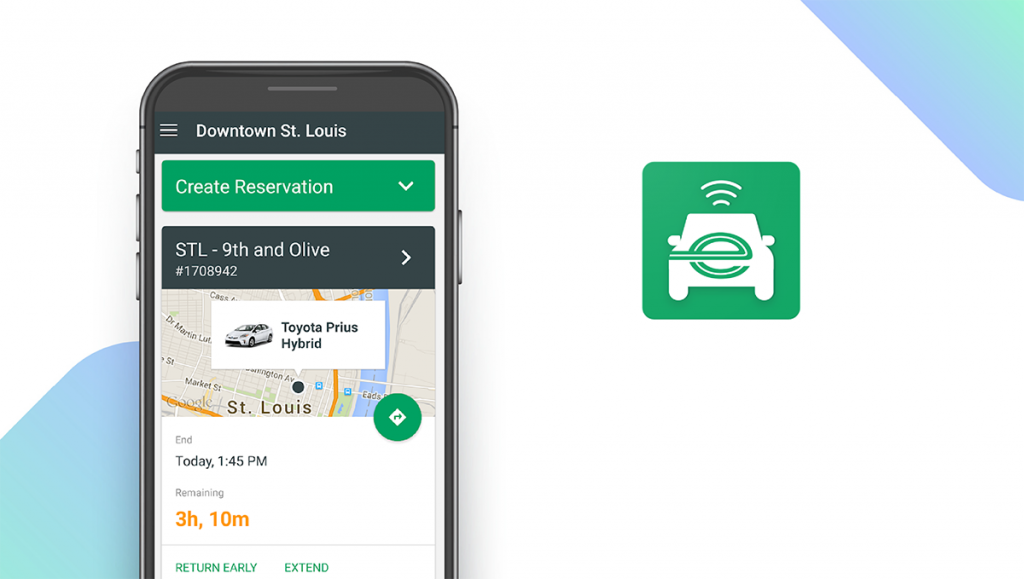In this image promoting Enterprise car rentals, the central focus is a white vehicle featuring the iconic green "E" logo of Enterprise. The green "E" is prominently displayed on the side of the car, which has Wi-Fi signal symbols emerging from its roof, signifying the vehicle’s connectivity features. The backdrop of the image is a gradient green-and-white, creating a clean and professional ambiance.

In the upper right corner of the image, there is a unique triangle shape. The top of the triangle points towards the top right corner, and the bottom right side is curved. This triangle displays a gradient transitioning from bright aqua blue at the top, through various shades, ending in periwinkle blue at the bottom.

Next to this triangle, there is an icon of a mobile phone showing three signal bars. The screen of the phone displays the text "Downtown St. Louis" next to a "Create Reservation" button with a drop-down menu. Below this, it reads "STL 9th and Olive" followed by a unique identifier "1708942" along with a greater-than sign, indicating additional details available upon selection.

The midsection of the image highlights a Toyota Prius Hybrid, depicted on what seems to be a map interface. The image of the Prius includes an arrow pointing down to St. Louis on the map. Below this, text indicates "End today at 1:45 PM, remaining 3 Hours and 10 Minutes," highlighted in orange. Following this, options "Return Early" or "Extend" are provided, with a navigational icon—a circle housing a right arrow inside a diamond—positioned on the right side.

Overall, the image seamlessly integrates various elements to showcase Enterprise's car rental services, connectivity, and convenient reservation features.